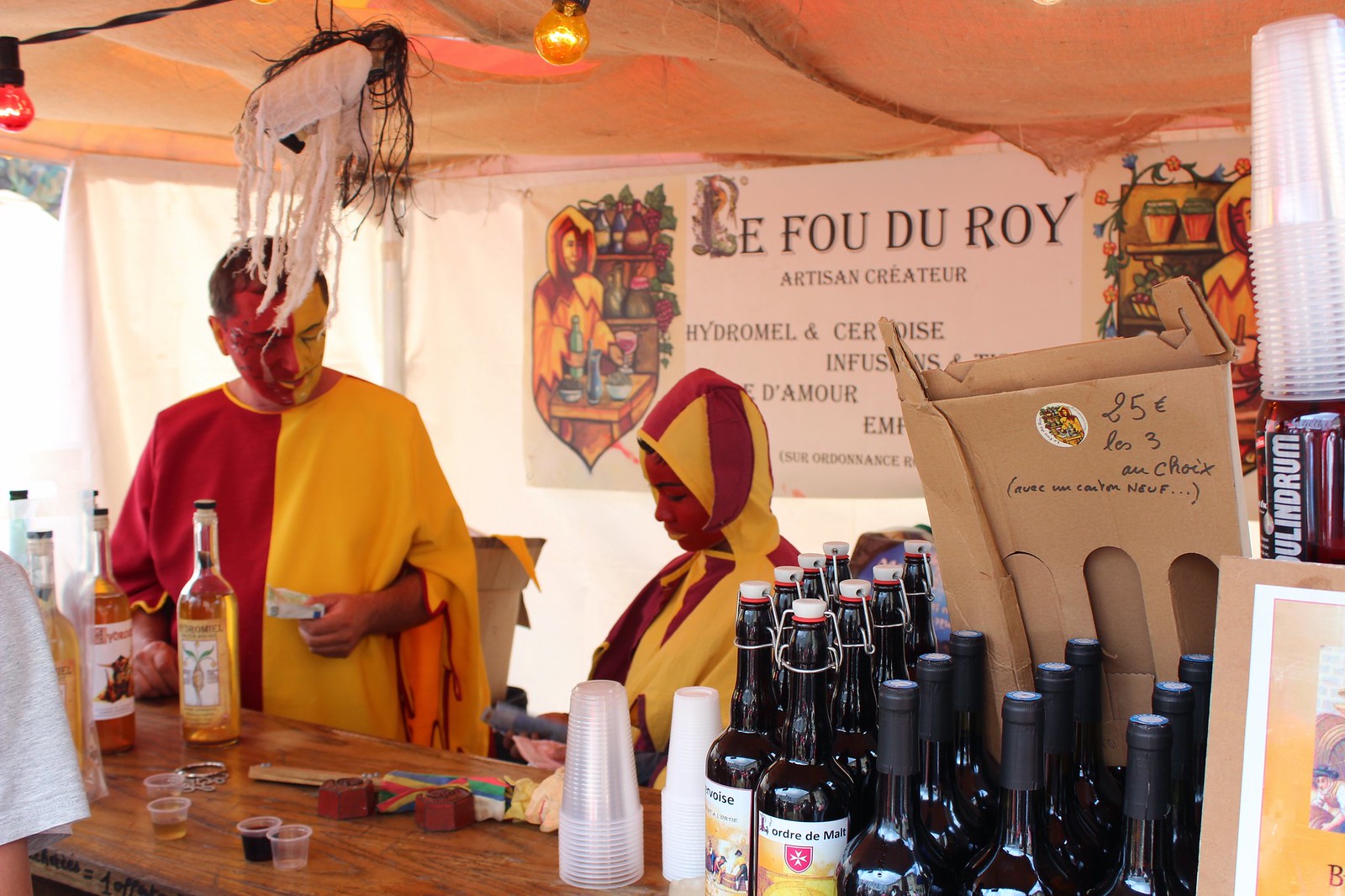The photo captures a vibrant festival stand, likely a tent, showcasing an array of artistic alcohol selections. At the center of the scene are two individuals, likely a man and a woman, donned in striking red and yellow outfits. Their costumes are uniquely designed with the left side red and the right side yellow, and their face paint mirrors this bold split. One of them also wears a matching yellow and red hood. They stand behind a brown table adorned with various bottles of alcohol; on the left, gold-colored bottles, and on the right, black bottles, possibly wine. Scattered on the table are sample cups and a stack of larger plastic cups beside a bigger bottle. Behind them hangs a sign reading "Le Faux Du Roy, Artisan Creator, Hydromel, Surroys Infusions," featuring imagery of individuals dressed similarly to the pair. The scene is illuminated by glowing red and yellow lights, contributing to the festive ambiance under the tan tent top.